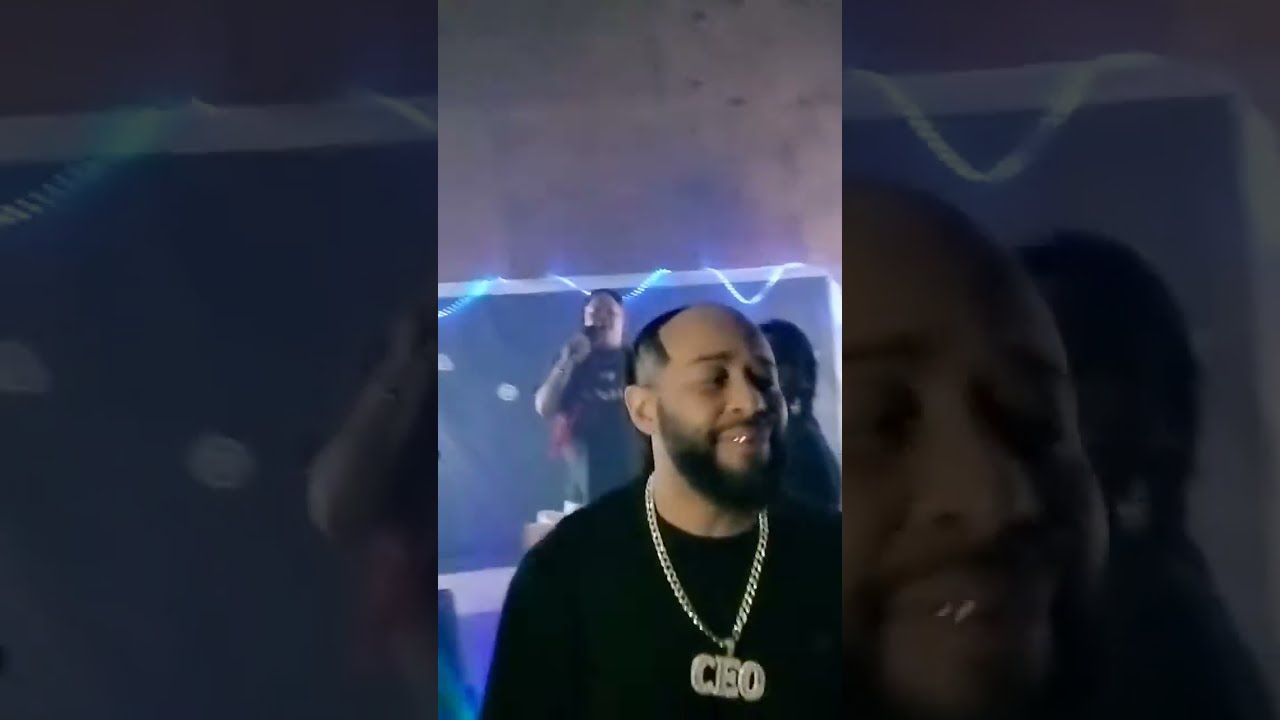In this high-definition photograph, the central figure is a man wearing a black shirt and a thick, gold necklace with a large "CEO" pendant. He has a dark-colored beard, a mustache, grills that appear to be gold, and a partially balding head. The image captures him in a club-like setting, as indicated by the smoky background and electric lights. 

Behind him, there is a performer on stage, holding a microphone and seemingly engaged in singing or rapping. The performer is also wearing a black shirt and has short hair. To the side of the stage, another person with long hair, possibly dreadlocks, is visible. The background features a mirror and stone-like walls, contributing to the club ambiance.

The photograph appears wider than it is tall and is divided into three sections. The central part, which is the focal point, is flanked by blurred, close-up border sections of the same scene, enhancing the depth and complexity of the image.